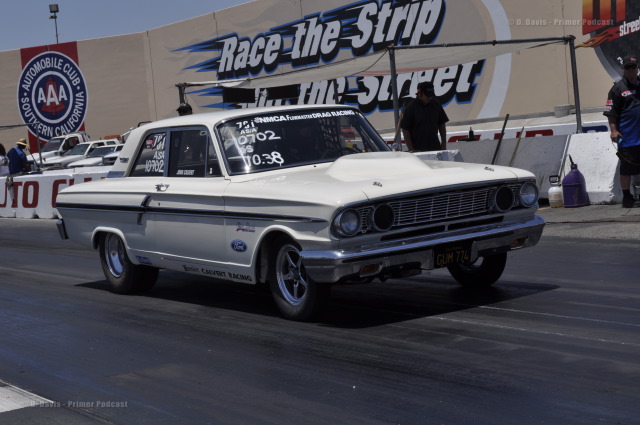This outdoor daytime image captures a nostalgic cream-colored muscle car, likely from the 1960s, racing down a track. The car, a vintage Ford, is adorned with various stickers and writing, including "NMCA Drag Racing" and numerous numbers on the windshield such as "0702 S10.3 8". Positioned on the dashboard are stickers with letter and number combinations, adding to its racing flair. The racetrack features protective barriers, with a prominent tan concrete barrier on the left that reads "Race the Strip" accompanied by blue streaks. Adjacent to this, there is a circular logo reading "Automobile Club Southern California AAA". The scene is bustling with activity, featuring a man in a straw hat and blue shirt, various white cars and trucks parked, and another individual beneath a white canopy, wearing a black cap and t-shirt, inspecting the ground. In the background, against a grey stone berm, multiple barrels and containers are visible. The upper corner of the image includes a watermark, "D Davis Primate Premiere Podcast," with "Street" also discernible, adding an extra layer of authenticity to this dynamic scene.